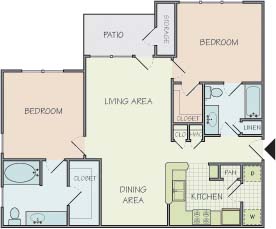This image depicts a detailed line drawing of a residential floor plan, possibly for an apartment or a house. The layout features two bedrooms, both highlighted in pink. A distinctive purple-colored patio extends from the living space, complete with an adjoining storage building. 

The central area of the home, which includes the living room, dining room, and a hallway, is shaded in light green. The kitchen is strategically placed near the entrance doorway, and a bathroom is situated directly across from the kitchen. Uniquely, this bathroom provides two access points: one leading to the smaller bedroom, and the other connecting to the living room.

The smaller bedroom, which can be reached either through the bathroom or the living room, also boasts a walk-in closet. Similarly, the second bedroom, located opposite the living and dining areas, features an expansive main bathroom with additional space and a walk-in closet situated within the bathroom itself. The smaller bedroom's bathroom has a dedicated linen closet. The hallway contains another closet, although a washer and dryer area is noticeably absent in the kitchen.